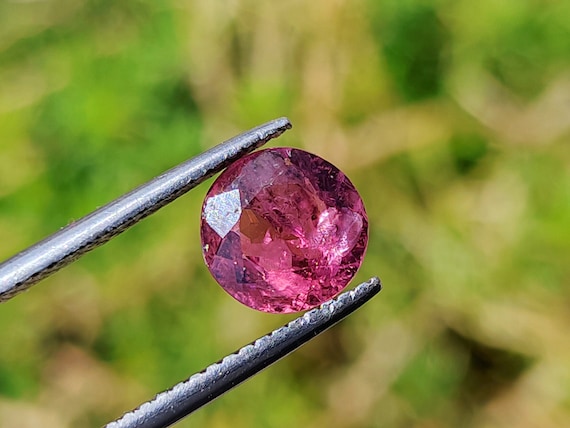This photograph features a striking image of a circular, dark pink gemstone held delicately by a pair of silver tweezers emerging from the bottom left corner of the frame. The gemstone, which appears to be a polished and possibly rough-cut diamond, is positioned centrally within the composition, showcasing its sparkling, multifaceted surface. The background is characterized by a blurry expanse of green, suggesting a natural, leafy, or grassy setting, which creates a vivid contrast with the jewel's vibrant hue. The absence of any other objects or people ensures that the viewer's attention remains focused on the gleaming gemstone and the precise grip of the metal tweezers holding it.